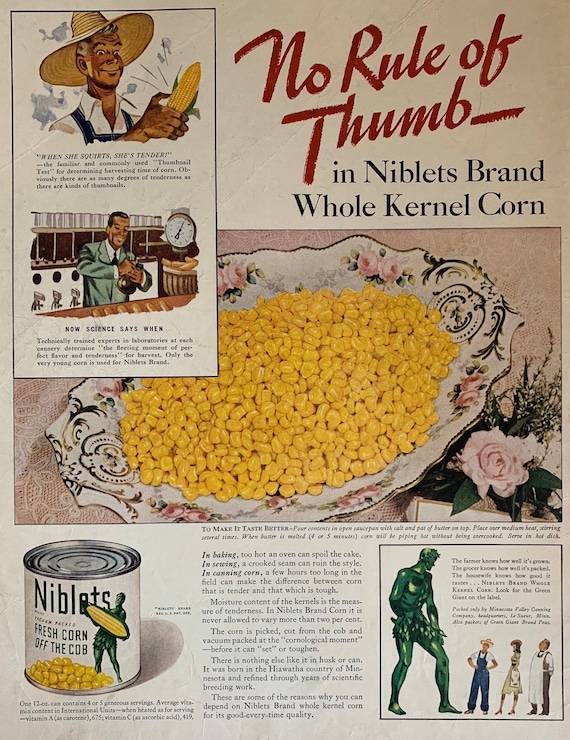This detailed advertisement from a vintage magazine promotes Green Giant's Niblet's brand whole kernel corn and features nostalgic, cartoon-style illustrations reminiscent of the 1960s. The advert, mostly dominated by text and images on the right, boldly declares "No Rule of Thumb" in red cursive script. On the left, a cartoon farmer, clad in a hat, holds an ear of corn near an inscription that reads, "When she squirts, she's tender." Below this, a smaller text elaborates, with phrases like "now science says, when," though much remains unreadable.

Centrally, a large casserole dish brims with plain white corn, emphasizing the product's wholesome simplicity. Beneath this dish, a can labeled "Niblet's Fresh Corn Off The Cob" showcases a green character, holding kernels of corn downward, likely representing the iconic Green Giant. This central can is flanked by more text, touching upon themes like baking, sewing, and canning.

On the lower right, a towering green figure unmistakably represents the Jolly Green Giant, gazing benevolently at a farmer, a woman, and a baker—all drawn much smaller than the giant himself. Meanwhile, on the right side of the advertisement, another farmer weighs corn in front of a grocery store scale, highlighting the product's farm-fresh authenticity.